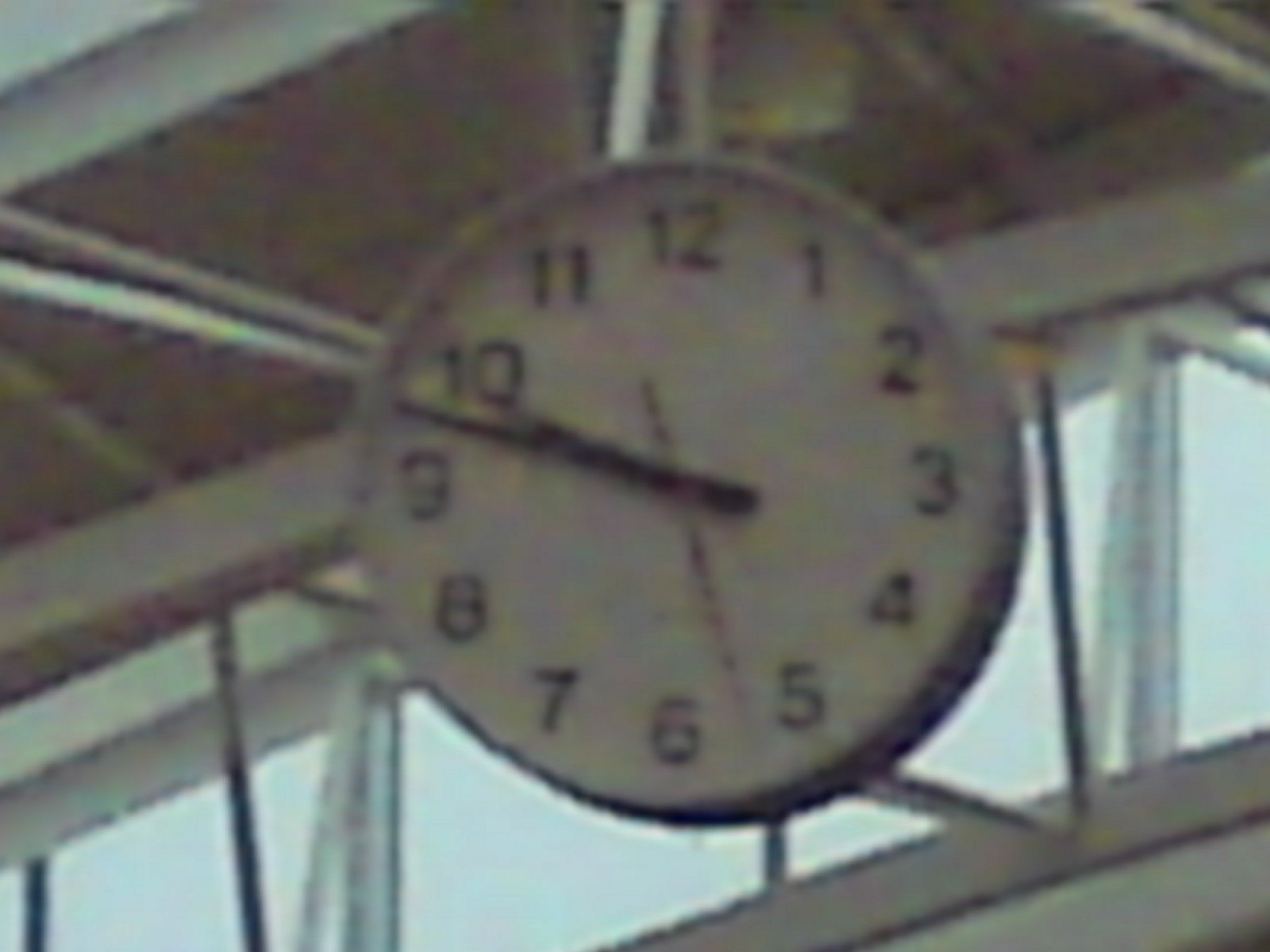In the center of the image is an intricate clock face with silver outlines around its edges. The clock is meticulously detailed and features numerals from 1 to 12. The second hand is pointing to 25 seconds, the minute hand is at 9, and the hour hand rests at 10. The face of the clock is white, providing a stark contrast to its metallic features. The background of the image is equally detailed, depicting a grey, overcast sky visible through large windows with metal bars and dividers. These architectural elements create an industrial ambiance, highlighted by the dark ceiling and the silver and grey hues that frame the scene. The connecting metals and structural supports add a sense of solidity and permanence to the clock's placement within this mysterious, possibly abandoned space.